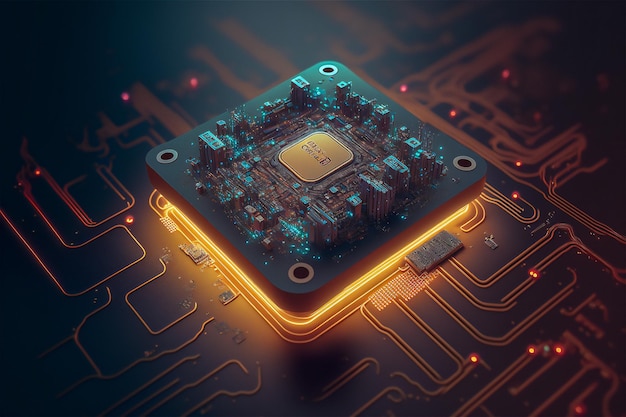The digital art image depicts a detailed electronic chip, prominently featuring a central, elevated square area. This raised section emits a yellowish light, illuminating the chip's intricate circuits and wires, which are yellow with scattered red dots. The design resembles a miniature cityscape, with interconnected components akin to buildings or skyscrapers. The chip, looking embedded in a potentially active, powered-on motherboard, showcases four distinct holes at the corners of the square area. Its backdrop is predominantly black, highlighting the glowing circuits and complex wiring. The portrayal is so precise it echoes the meticulous construction facilitated by modern robotics in electronics manufacturing.